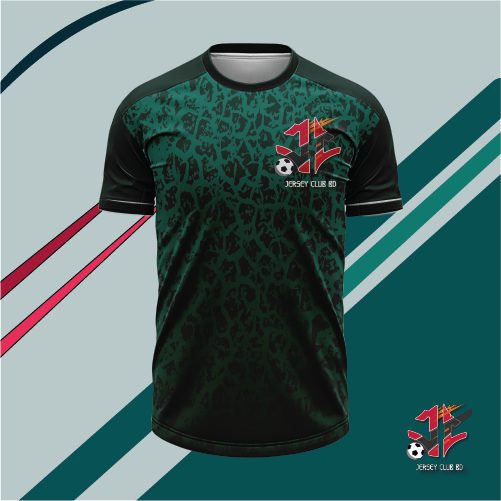The image showcases a detailed, short-sleeved football jersey, primarily featuring a blend of dark and light green hues in a checkered or camo-like pattern. The front of the jersey is a lighter green with a dark green, animal-print-inspired motif, while the back is a solid dark green. The shoulders and sleeves are a darker blue, adding contrast to the design. Adorned on the right chest is a red branding logo that includes a small, difficult-to-discern red design. The logo also features a small soccer ball and the text "Jersey Club BD" beneath it. The background of the image consists of diagonal stripes in shades of teal, light green, and dark green, with additional dynamic orange or red slashes contributing a sense of movement, enhancing the jersey's promotional composition. At the bottom right corner of the background, the Jersey Club BD logo is repeated, tying the theme together visually. This image appears to be part of an advertising campaign by Jersey Club BD.